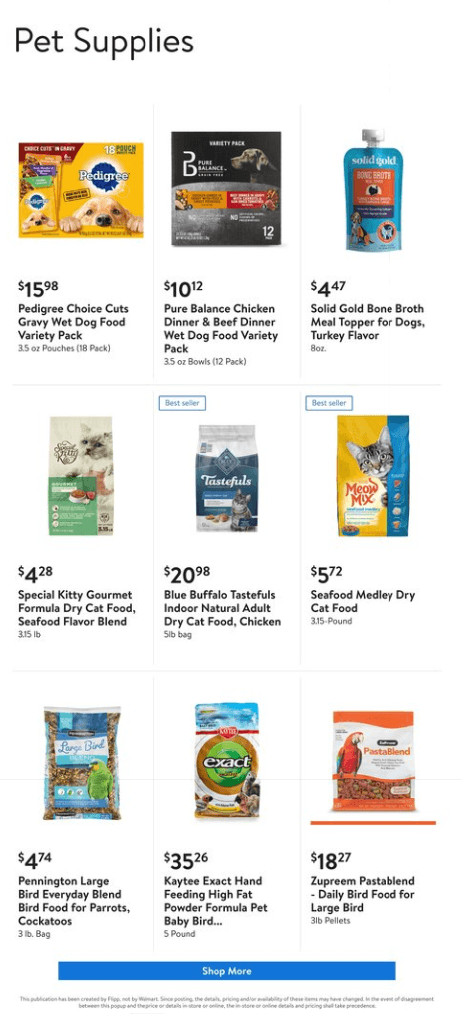**Detailed Caption:**

This image captures a section of a shopping website dedicated to pet supplies, arranged in a 3x3 grid layout displaying nine different product options. 

- **Top Row:**
  1. **Top Left:** A package of Pedigree Choice Cuts in Gravy wet dog food.
  2. **Center Left:** A black box containing a Pure Balance Chicken Dinner and Beef Dinner wet dog food variety pack.
  3. **Top Right:** A yogurt-like pack labeled Solid Gold Bone Broth Meal Topper for Dogs, Turkey Flavor.

- **Middle Row:**
  4. **Middle Left:** A green and white bag of Special Kitty Gourmet Formula dried cat food.
  5. **Center Middle:** A white and blue bag of Blue Buffalo Tastefuls Indoor Natural Adult Dry Cat Food with Chicken, tagged as a bestseller.
  6. **Middle Right:** Another bestseller, a yellow and blue bag of Seafood Medley dry cat food.

- **Bottom Row:**
  7. **Bottom Left:** A bag labeled Pennington Large Bird Everyday Blend Bird Food for parrots and cockatoos.
  8. **Center Bottom:** A white bag with a green circle, containing Kaytee Exact Hand Feeding High Fat Powder Formula for baby birds.
  9. **Bottom Right:** A red and white bag featuring the image of a parrot, labeled Supreme Pasta Blend Daily Bird Food for large birds.

At the very bottom of the grid, there is a prominent blue rectangular button that invites users to "Shop for More".